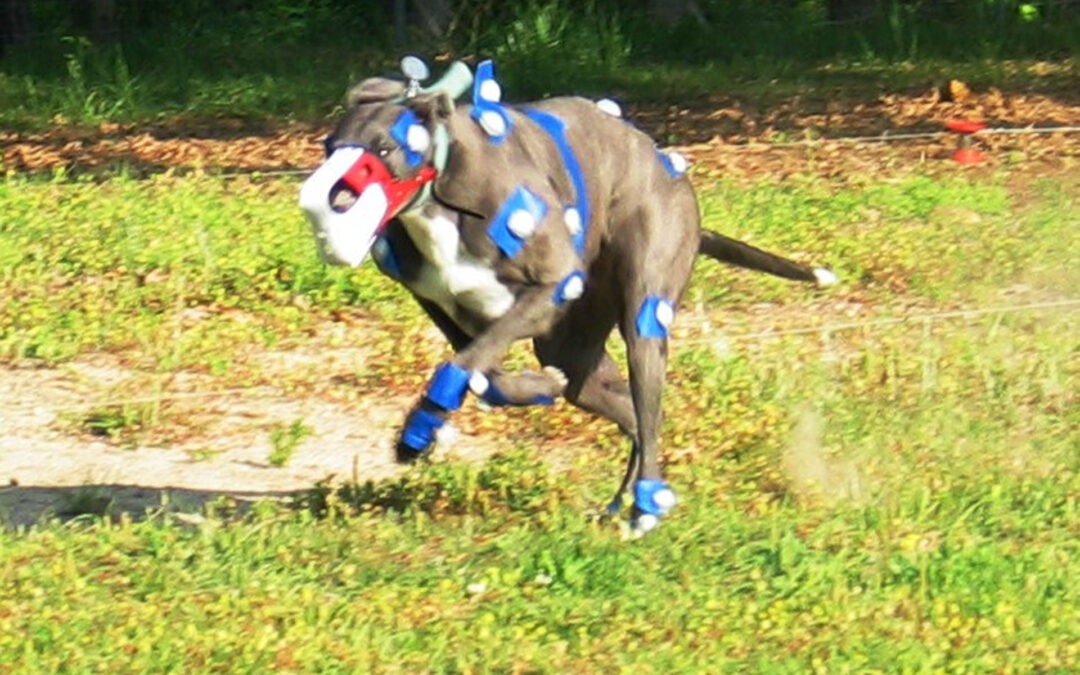The image depicts an outdoor, daytime scene featuring a dog mid-air, possibly captured while running on a patch of green-yellow grass. Despite the overall blurriness and low quality of the image, several details are clear. The dog, with a dark gray coat and white patches below its neck, is adorned with multiple blue motion capture (mocap) stickers, each with a white circular center—strategically placed on its legs, body, and head. The dog is also wearing a red and white muzzle, reminiscent of those used on racing greyhounds. The background consists predominantly of green grass with hints of brown, suggesting varying grass health and sunlight intensity. The bright setting underlines the clear daytime conditions.